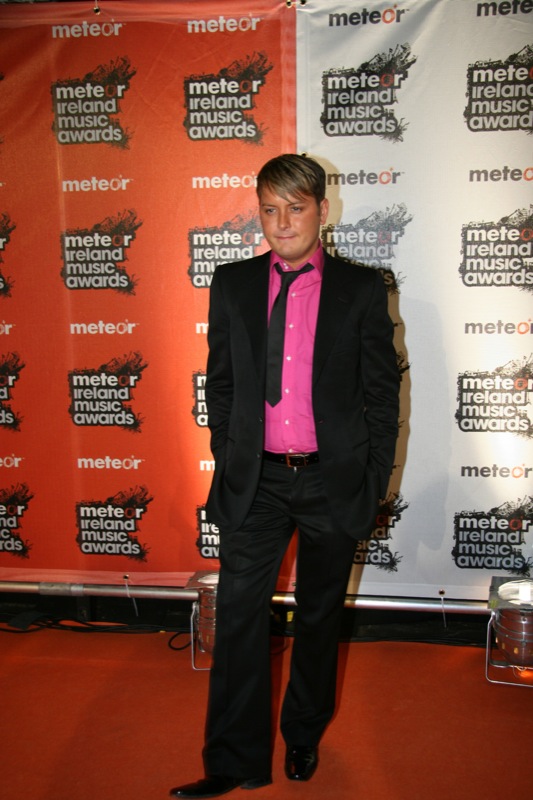This color photograph captures a young individual, possibly a celebrity, standing alone on an orange carpet at the Meteor Ireland Music Awards. The backdrop of the image features an orange and white banner repeatedly displaying the event's name. The person, positioned centrally, is dressed in an elegant ensemble consisting of black shoes, pants, belt, jacket, and tie, complemented by a bright pink button-down shirt. They are Caucasian, with very short brown hair highlighted with blonde streaks at the front, and their left ear is visible. Though the individual's gender is not apparent, their detailed attire and the prominence of large silver spotlights aimed upward in the background add to the glamour of the awards show setting. A shadow cast on the white portion of the banner and the overall indoor ambiance enhance the photograph's sophistication.